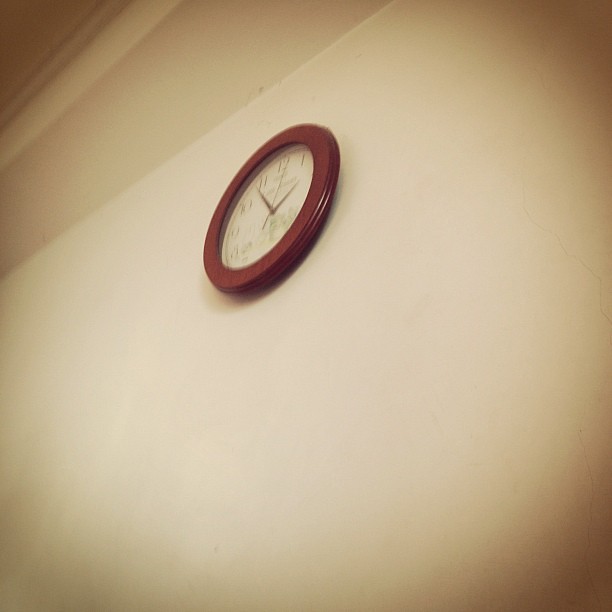This blurred, color photograph captures an indoor setting with a focus on a beige wall adorned by a round clock. The shot is angled upwards, drawing attention to the clock placed centrally on the wall. The wall is primarily a beige hue, with a subtle, darker beige line running above the clock. The image features shadows, particularly at the bottom left, right, and upper right, with a distinct orange tint. In the upper left corner, slanted beams are faintly visible, contributing to the composition of the room.

The clock, which serves as the centerpiece, boasts a red exterior rim. Soft light illuminates the right side of the clock's face, enhancing its visibility against the wall. The clock features black numerals that are barely discernible due to the image's blurriness. Its thin black hour and minute hands, along with a possibly even thinner black second hand, indicate the time as approximately five minutes to two. A slight shadow cast directly beneath the clock adds to the depth and dimension of the photograph.